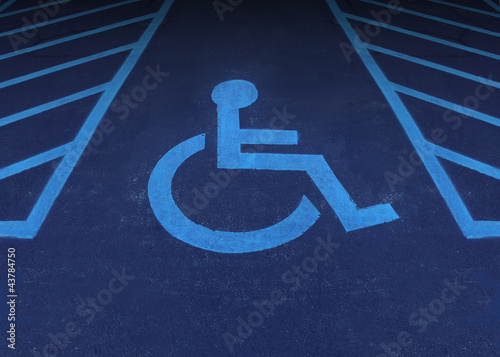This image captures a nighttime aerial view of a freshly paved handicap parking space in a parking lot. The ground is a dark asphalt, appearing brand new, with the boundaries of the space clearly marked. The center of the image prominently features the universally recognized handicap symbol - a stick figure seated in a wheelchair - painted in a lighter shade of blue against a dark blue background. Flanking this symbol on both the left and right are rectangular sections filled with diagonal lines, indicating no-parking zones. The edges of the photograph appear slightly darker, enhancing the central focus on the parking space. Additionally, small vertical text, bearing the watermark "Adobe Stock," is superimposed along the bottom left and right corners of the image. The color palette is limited to black, white, and various shades of blue, emphasizing the designated parking area's details.